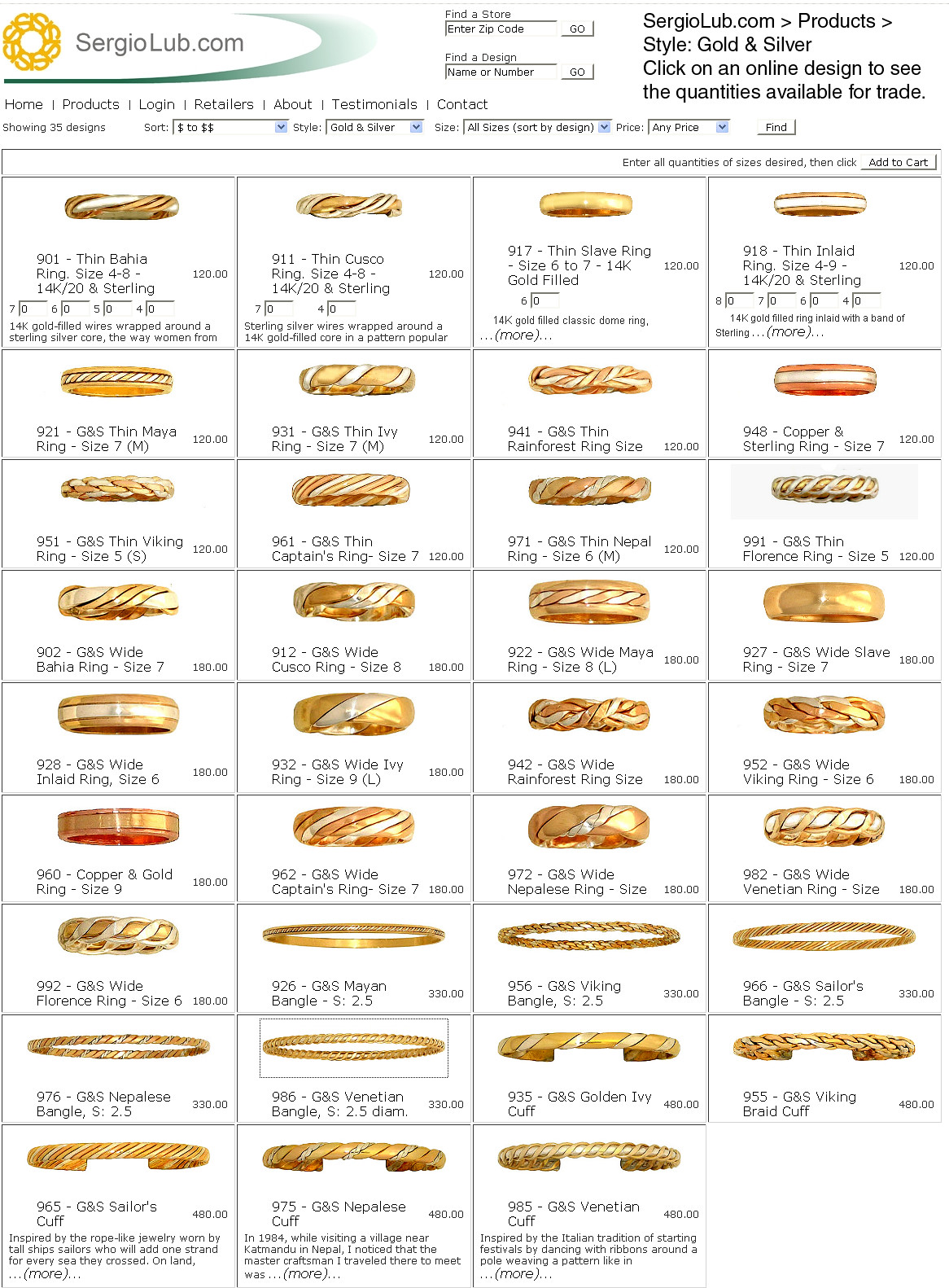This is an image of a webpage advertisement from SergioLUB.com, showcasing a selection of gold wedding bands and rings against a white background. The banner at the top prominently displays "SergioLUB.com" along with navigational options such as "Find a store, enter zip code, find a design, name or number". Various categories like "products, style, gold and silver" are accessible, and there's functionality to sort designs based on price ranges or specific criteria by inputting desired specifications.

The image includes 35 different ring designs, details of which are meticulously listed. Each ring is labeled with a product identification number like "961-GNS" and is accompanied by a descriptive name—for instance, "Thin Captain's Ring Size 7" and "Wide Viking Ring Size 6". They also display prices, with most rings spanning from $120 to $180, although some adorned with diamond baguettes exceed $400.

Additionally, the rings are segmented by style, including thin and wide bands, along with some special designs such as "Thin Bahia Ring", "Thin Cusco Ring", and "Wide Ivy Ring". The image encapsulates the variety offered, enhancing the viewer’s experience by showcasing detailed product names, sizes, and prices all neatly organized for potential shoppers.